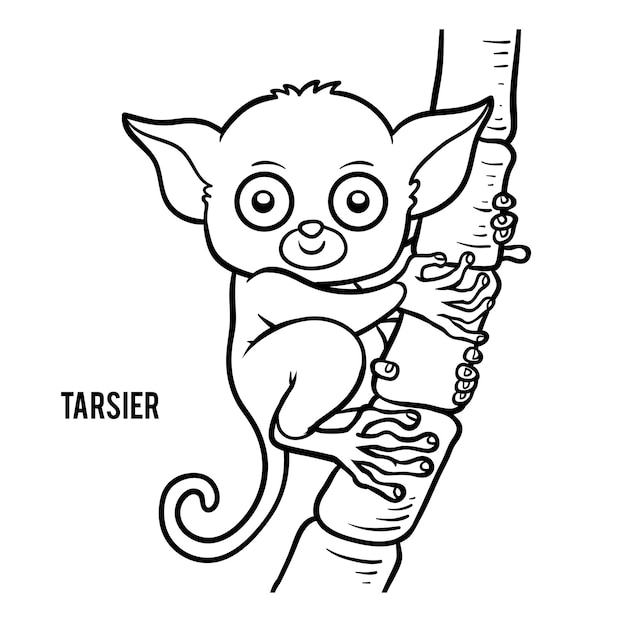This is a detailed black-and-white ink drawing of a tarsier, prominently displayed against a stark white background. The artist's name is inscribed to the left of the drawing, and in bold, all-caps lettering, the word "TARSIER" is clearly visible. The tarsier is depicted clutching what appears to be a bamboo tree trunk or limb with its small, detailed feet and hands. Its head is roundish with large, expressive eyes and long ears that jut out to the sides, contributing to its endearing appearance. The creature's nose is a cute button shape, and below it, a subtle smile adds to its charm. Its body is rather stubby, and a long, curled tail suggests a sense of contentment. Some fine details include four visible toes on one foot and four or five fingers on one hand, all meticulously represented in the illustration. The overall scene captures the tarsier gazing directly at the viewer with a delighted expression, making for an engaging and heartwarming composition.